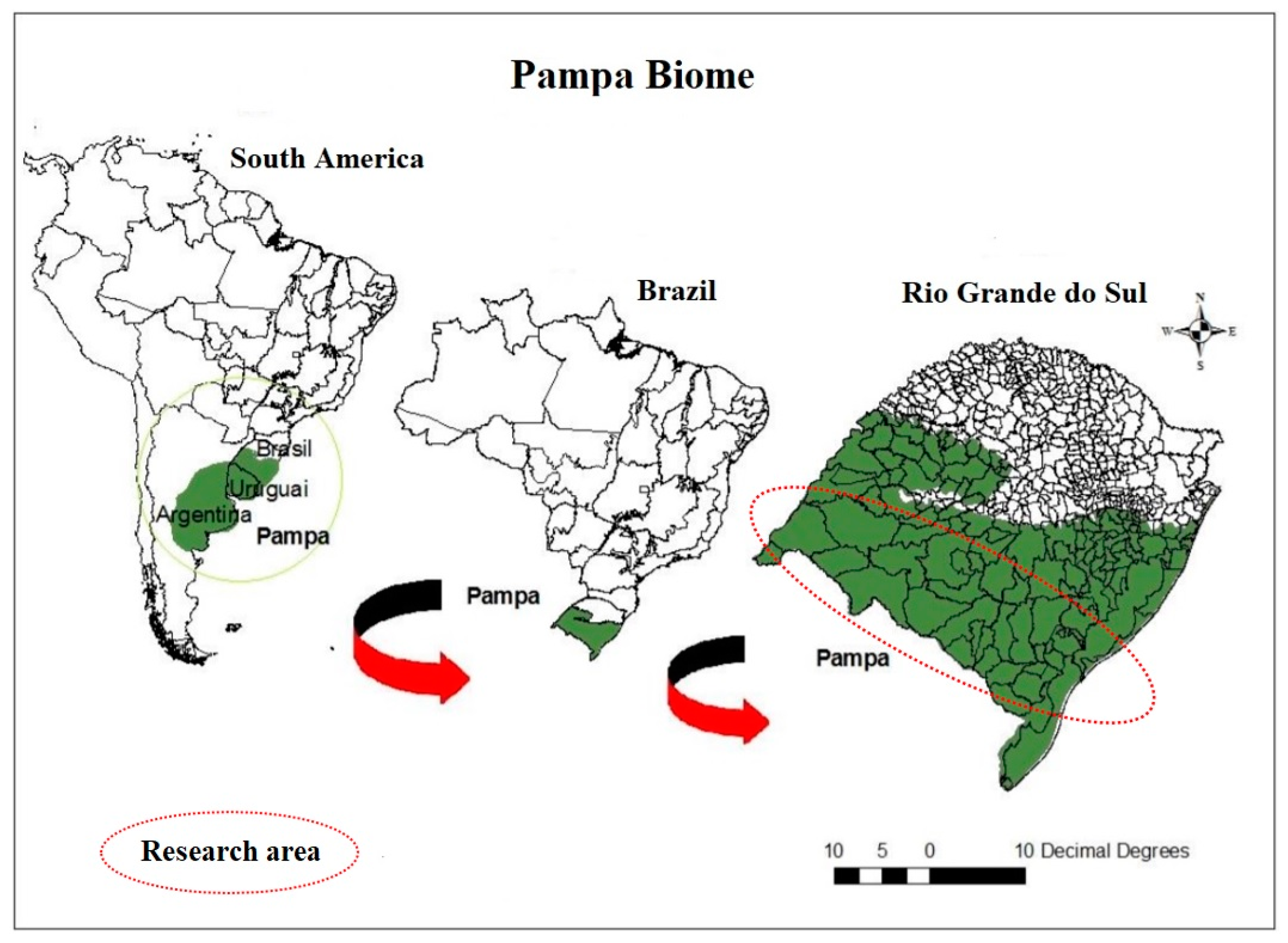The illustration depicts three side-by-side maps of South America, Brazil, and Rio Grande do Sul, each outlined in black against a white background. At the top, the title "Pampa Biome" is prominently displayed in black text. On the left, the South America map highlights regions of Brazil, Uruguay, and Argentina in green, indicating the Pampa area. The central map focuses on Brazil with its southern tip marked in green, while the rightmost map zooms in on Rio Grande do Sul, displaying over half of the state in green. Each map features a red arrow pointing to the green area, labeled "Pampa."

At the bottom of the illustration, the left corner bears a red dotted oval encircling the term "Research Area," denoting a specific study region within Rio Grande do Sul. Additionally, a legend on the bottom right provides a scale in decimal degrees. A diamond-shaped compass appears to the right of the text, orienting north at the top. The entire visual effectively maps the extent of the Pampa biome across these geographic scales, with clear annotations and highlighted regions for easy reference.